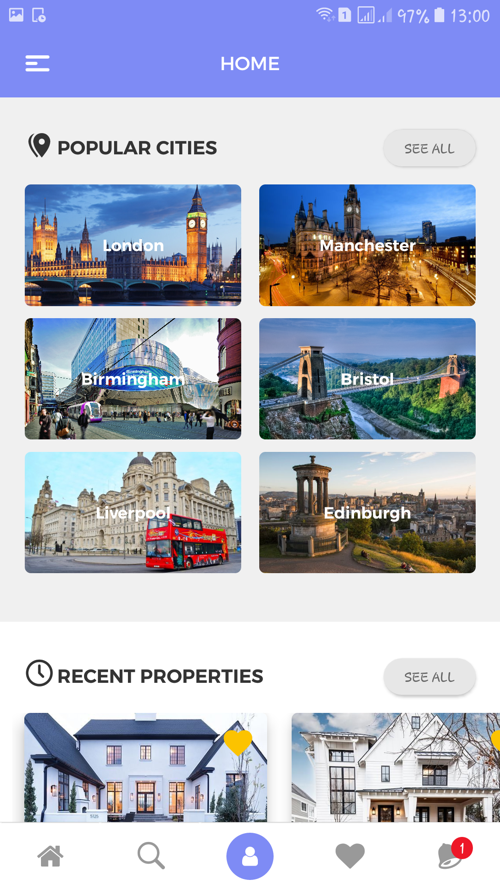The image is a detailed screenshot of a travel website. The webpage prominently displays several cities, each represented by distinctive cityscapes. At the top left of the screen, there is a blue home button with white text. The screen shows the status bar, indicating the carrier signal strength at two bars, Wi-Fi connectivity, the time as 1:00 PM, and the battery life at 97%.

Below the status bar, the header section features the title "Popular Cities" in black font against a gray background, accompanied by a pin icon. There is also a "See All" option next to this header. The cities showcased include:

- London: Depicted with a recognizable city backdrop.
- Manchester: Featuring an urban cityscape.
- Birmingham: Highlighted with a view of its city scenery.
- Bristol: Displayed with a large bridge, likely the Clifton Suspension Bridge.
- Liverpool: Shown with an iconic red double-decker bus.
- Edinburgh: Presented from a vantage point overlooking the city, providing a panoramic view.

At the bottom of the screen, there is a section for "Recent Properties," with another "See All" option available. The navigation bar at the bottom of the page includes icons for home, search (magnifying glass), profile, favorites (heart), and notifications (bell).